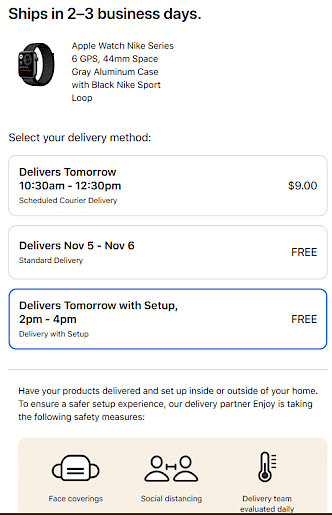This screenshot from an unidentified website displays detailed product and delivery information for an Apple Watch Nike Series 6 GPS 44mm in a space gray aluminum case with a black Nike sport loop. At the top, a banner announces, "Ships in two to three business days." The central image showcases a sleek black Apple Watch. 

Beside the photograph, product specifics and delivery options are outlined. Customers can select from multiple delivery methods: 

1. **Scheduled Courier Delivery**: Guaranteed delivery by 10:30 a.m. to 12:30 p.m. the next day for a fee of $9.00.
2. **Standard Delivery**: Expected arrival between November 5th and November 6th, free of charge.
3. **Delivery with Setup**: Complimentary next-day delivery between 2 p.m. and 4 p.m., including product setup.

This section is highlighted with a blue rectangle for emphasis. Detailed guidance follows about ensuring a safe delivery and setup experience. The delivery partner, Enjoy, adheres to strict safety protocols which include:

- **Face Coverings**: Illustrated by an icon of a face mask.
- **Social Distancing**: Depicted with an icon showing two people separated by a horizontal line.
- **Daily Health Evaluations**: Represented by a thermometer graphic.

The focus of the screenshot remains on the Apple Watch and the accompanying text, without any additional photographic elements, animals, birds, plants, flowers, or trees.